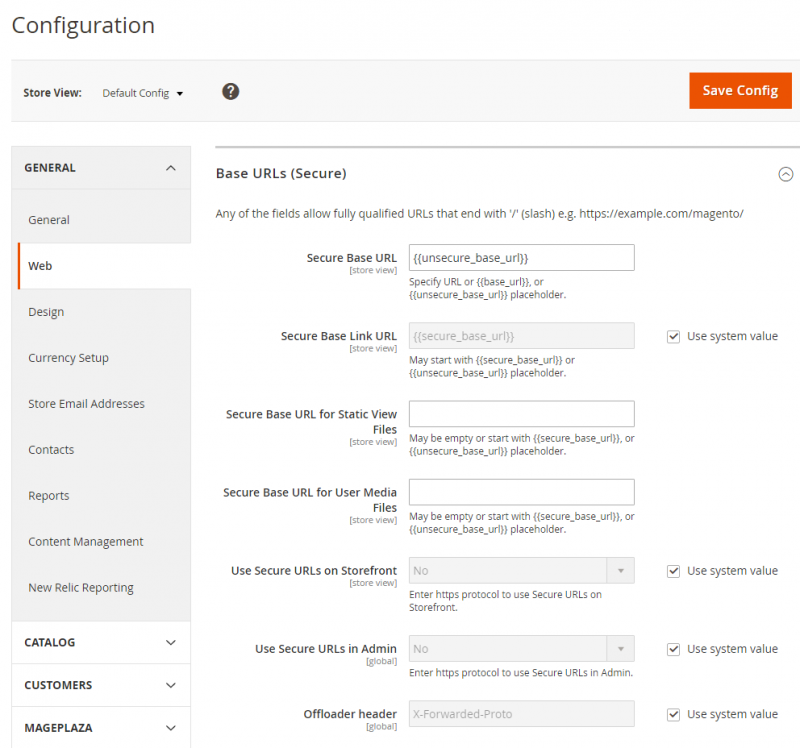The image depicts a configuration page within a specific website, program, or app, primarily featuring a white background. Prominently at the top, the title "Configuration" is displayed in a bold black font. Directly beneath this title, there is a light gray box containing the bolded text "Store Review" in black. Adjacent to this, the term "Default Config" appears in regular black font, accompanied by a black drop-down arrow indicating the availability of different options. To the immediate right, a black circle with a white question mark icon suggests an area where users can obtain additional information. 

On the far right side of the page, an orange box with white text is labeled "Save Config." 

Below this header section, on the left-hand side, a white background features a menu with various options under the "General" category, including "General," "Web," "Design," "Currency Setup," "Store Email Addresses," "Contacts," "Reports," "Content Management," and "New Relic Reporting." Additionally, broader categories such as "Catalog," "Customers," and "Match Plaza" are presented.

The selected option is "Web," revealing a detailed section where users can modify various web-related settings. The subsection heading "Base URLs (Secure)" is highlighted, presenting editable fields for the secure base URL and the secure base link URL, among other details. Users have the option to check a box to use the system value for each setting, allowing for further customization and configuration adjustments.